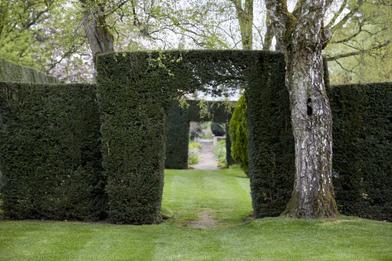The image depicts a lush, green garden, dominated by a striking archway meticulously shaped out of dense, dark forest green hedges that serve as a natural doorway. Surrounding this main arch are additional hedges that create a wall-like structure. To the right of the archway stands a tall, gray-brown tree with ashy-colored bark, adding to the natural feel of the scene. Beyond the initial arch, you can see a secondary archway in the distance, enhancing the garden's depth and symmetry. The ground is covered in freshly cut, lighter lime green grass with visible mowing lines and a worn pathway leading straight through the arch. In the background, numerous trees with abundant green leaves contribute to the overall verdant setting, with the sky appearing almost white. The arch itself has a thickness discrepancy, being thicker on the left side with some sparse areas at the top where the leaves do not fully cover. Overall, the scene is a beautifully maintained, natural outdoor space with a peaceful, inviting atmosphere.